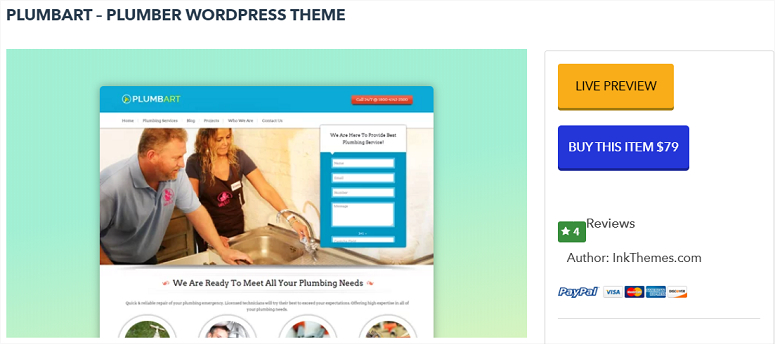The image features a wide rectangular design with a pastel green background that gradients to a lighter, yellowish-green at the bottom. Overlaying this background are bold, uppercase black letters spelling out "PLUMBART - Plumber WordPress Theme."

Within the green border sits a nearly square inner rectangle. The upper portion of this inner rectangle includes a medium blue banner which reads "Plumbart" on the left and has a wide, narrow red rectangle with white letters on the right. Just below this, a white banner displays menu items from left to right.

Beneath the white banner is a rectangular photograph. On the left side of the image, a man wearing a gray short-sleeve shirt with a red logo stands next to a woman on the right, who is dressed in a gray v-neck short-sleeve t-shirt. Adjacent to the woman on the right, a blue and white square appears, possibly indicative of a form field, with white lines inside it. The woman, with light brown hair cascading below her shoulders, reaches her left arm towards a sink faucet. The man leans over the sink, observing her actions.

Below this main picture, in black lettering, are the words: "We are ready to meet all your plumbing needs." Further down, a line of finer print runs from left to right, but it is not legible. At the bottom of the image, there are four half-circle images with white borders, aligned horizontally. From left to right, the first half-circle shows some green, the second one displays the top of a man's head, the third features gray and red colors, and the last half-circle presents shades of light brown and orange.